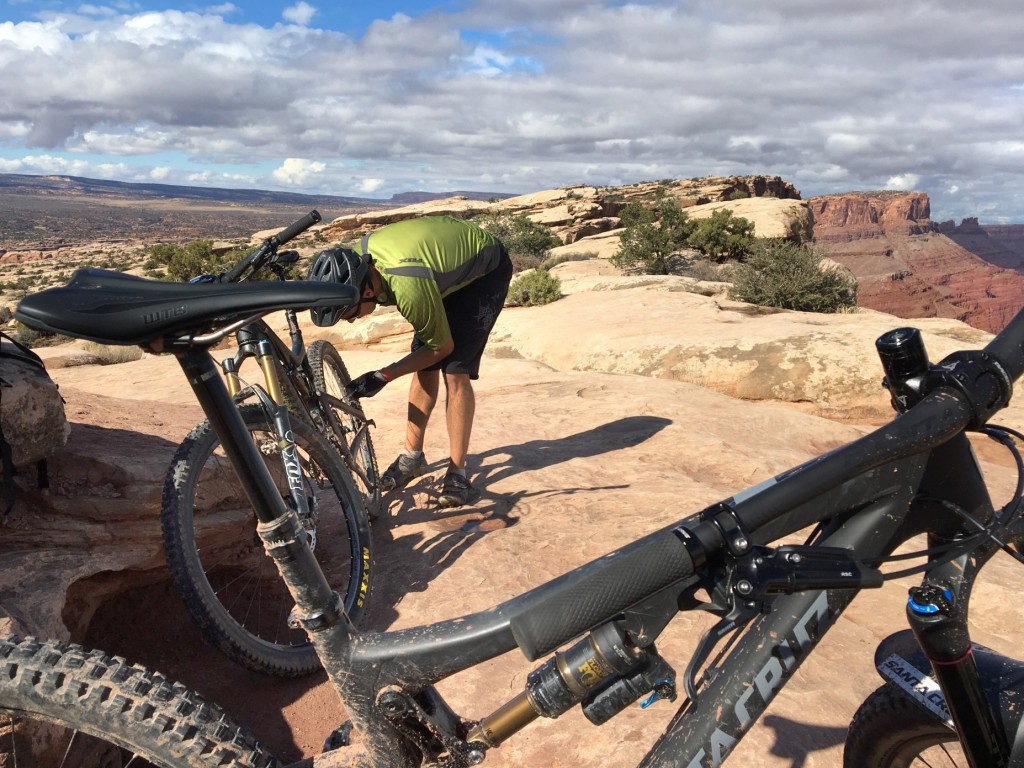This full-color photograph captures an outdoor scene on a cloudy day, utilizing natural sunlight. The image is nearly square with the sky taking up the top portion, showing heavy clouds with patches of blue, and stretches down to the rocky horizon. The setting appears to be a high-altitude, rocky desert area, possibly in Nevada or Utah. Dominating the bottom of the picture is a parked black mountain bike with a thin seat and a notably large back tire, but no rider.

Slightly left of center, a white male biker is performing maintenance on another bicycle. He is geared up in a black helmet, green shiny shirt, black shorts, gloves, and dark-colored shoes. The rocky surface they stand on is flat, with some reddish rocks and sparse shrubbery visible. Despite the overcast sky, the scene is vividly lit, highlighting the ruggedness of the terrain and the details of the bikes and their gear. This high-altitude plateau showcases the vast, dramatic landscape, emphasizing the sport of mountain biking amid nature's raw beauty.